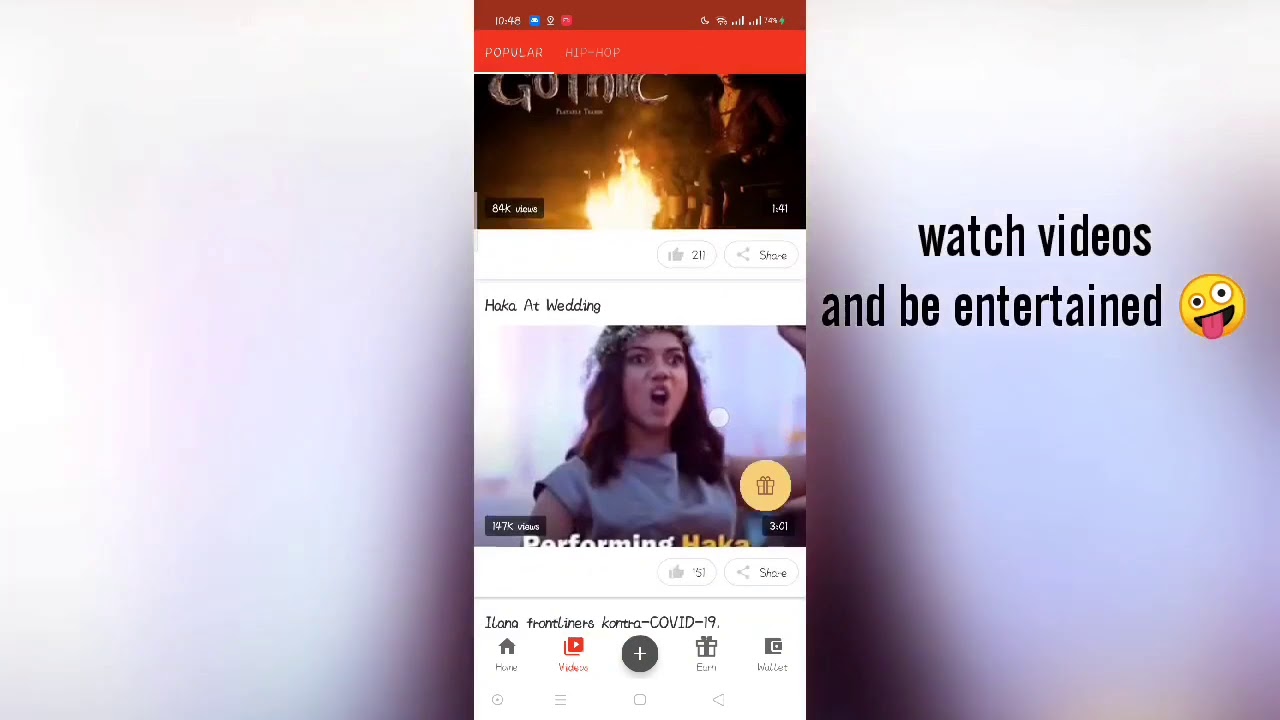The image displays a superimposed cell phone screen against a white background. On the right side of the screen, there's a playful message saying "Watch videos and be entertained," accompanied by a quirky smiley face with one larger eye and its tongue sticking out. At the top of the cell phone screen, the time is shown as 10:48, alongside cell reception bars.

The page features a red banner labeled "popular" with categories such as Hip Hop and Gothic. The text under Gothic is too small to read clearly due to low resolution, but it mentions 84,000 views for a video that is 1 minute and 41 seconds long, with 20 likes. Below this, there is a video titled "HAKA at wedding" with 147,000 views and a duration of 3 minutes and 1 second. This video has a yellow circle icon with a present box symbol and has received 51 likes, accompanied by a share button.

Further down, there is text reading "Ilana Frontliners KONTIA COVID-19," likely referring to content related to frontline workers during the COVID-19 pandemic.